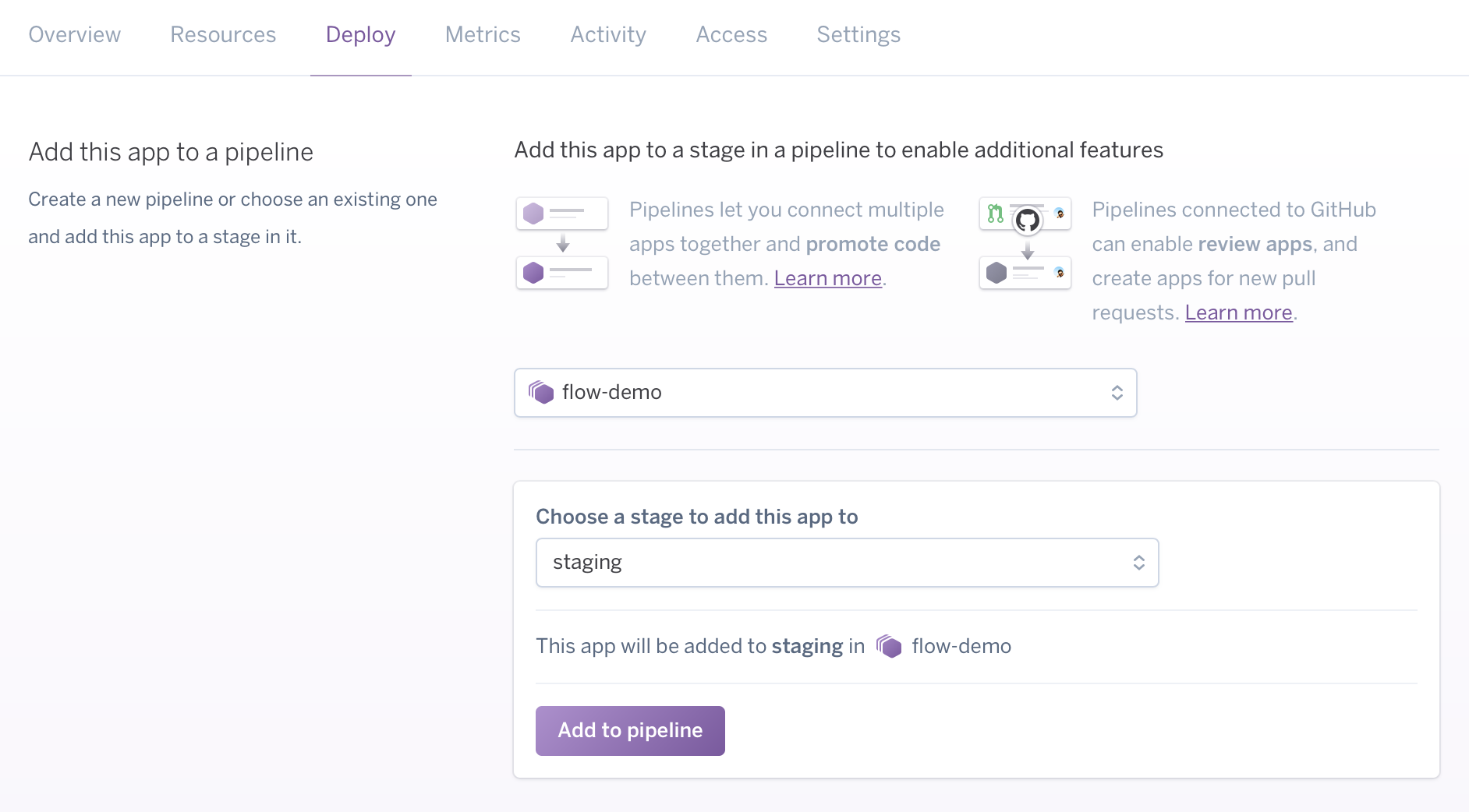The image appears to be a screenshot from a web page, possibly from GitHub. The top navigation bar includes selectable options presented from left to right: "Overview," "Resources," "Deploy," "Metrics," "Activity," "Access," and "Settings." The "Deploy" option is highlighted in purple, indicating it is currently selected, while the other options remain in gray.

Beneath this navigation bar, there is a solid gray line. Below this line, on the left side of the screen, there's text that reads: "Add this app to a pipeline." Underneath this heading, it further explains, "Create a new pipeline or choose an existing one, and add this app to a stage in it."

On the right side, there's additional text saying: "Add this app to a stage in a pipeline to enable additional features." Below this text, there is a small purple icon within a rectangular box that contains the message: "Pipelines let you connect multiple apps together and promote code between them," along with a link to "Learn more."

Further down the page, there's a prominent long rectangle labeled "Flow Demo." Below this, there is a large rectangular box prompting the user to "Choose a stage to add this app to," with a dropdown box labeled "Staging." Another line of text confirms: "This app will be added to staging in flow demo."

At the bottom, there's a purple rectangle button with white lettering stating "Add to Pipeline."